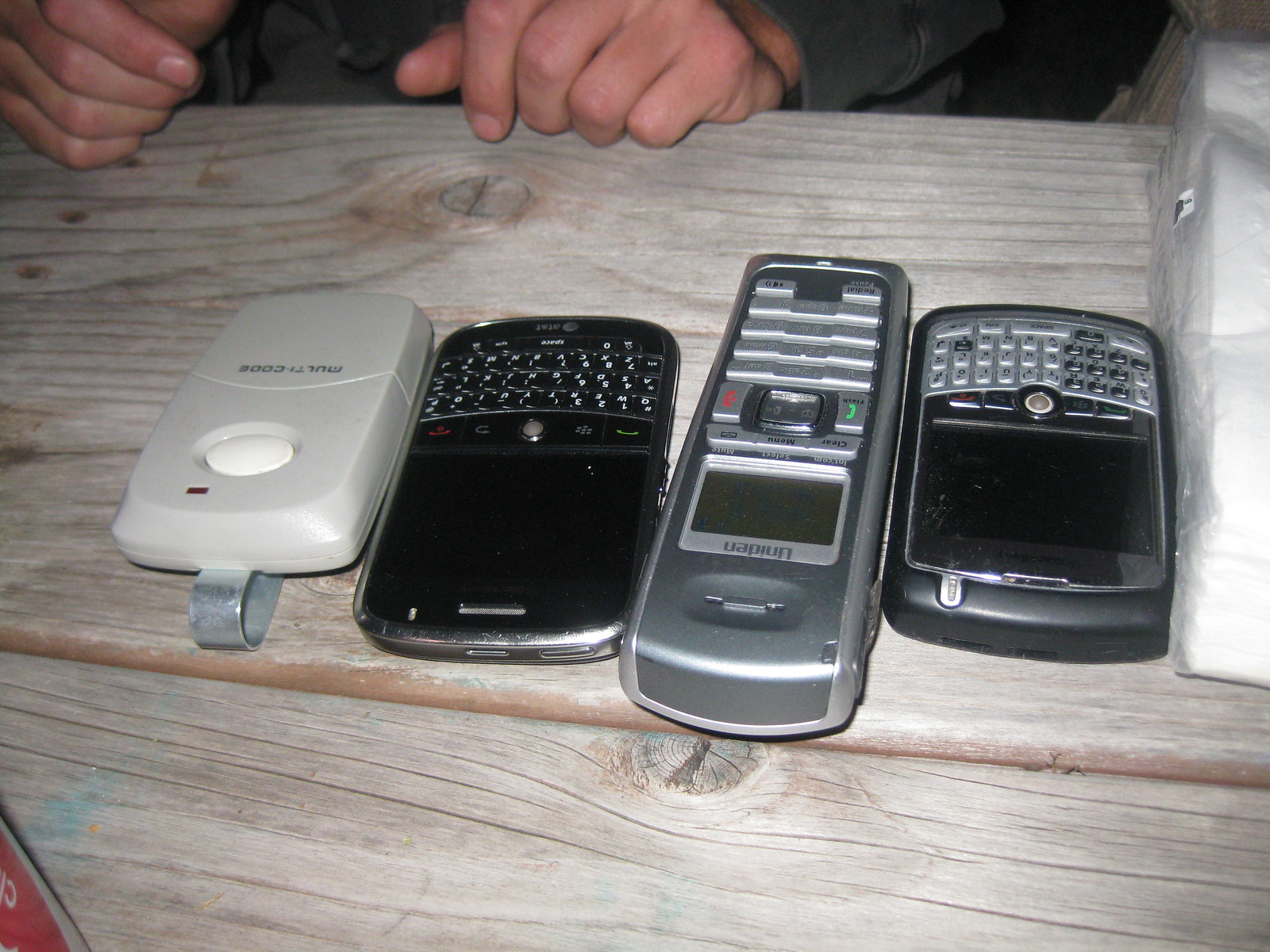The image captures an aged light grayish-brown wooden tabletop, likely a picnic table. Positioned on the table are four devices. On the far left is a white flip phone or garage door opener with a large white button and a silver clip curling underneath it. Next to it is a black BlackBerry phone with a keypad on the front. The third device is a silver and dark gray Uniden cordless phone, recognizable by the buttons on its lower half. The last device to the right is another black BlackBerry phone, this one featuring a gray keypad area. The devices are oriented with their screens at the bottom of the picture and their bottoms at the top. Above the devices, in the top part of the image, there is a pair of hands visible, wearing a gray shirt. To the right side of the image, a piece of white fabric or napkin is noticeable. A hint of red with white text can be seen at the bottom left corner of the image, adding a splash of color to the scene.